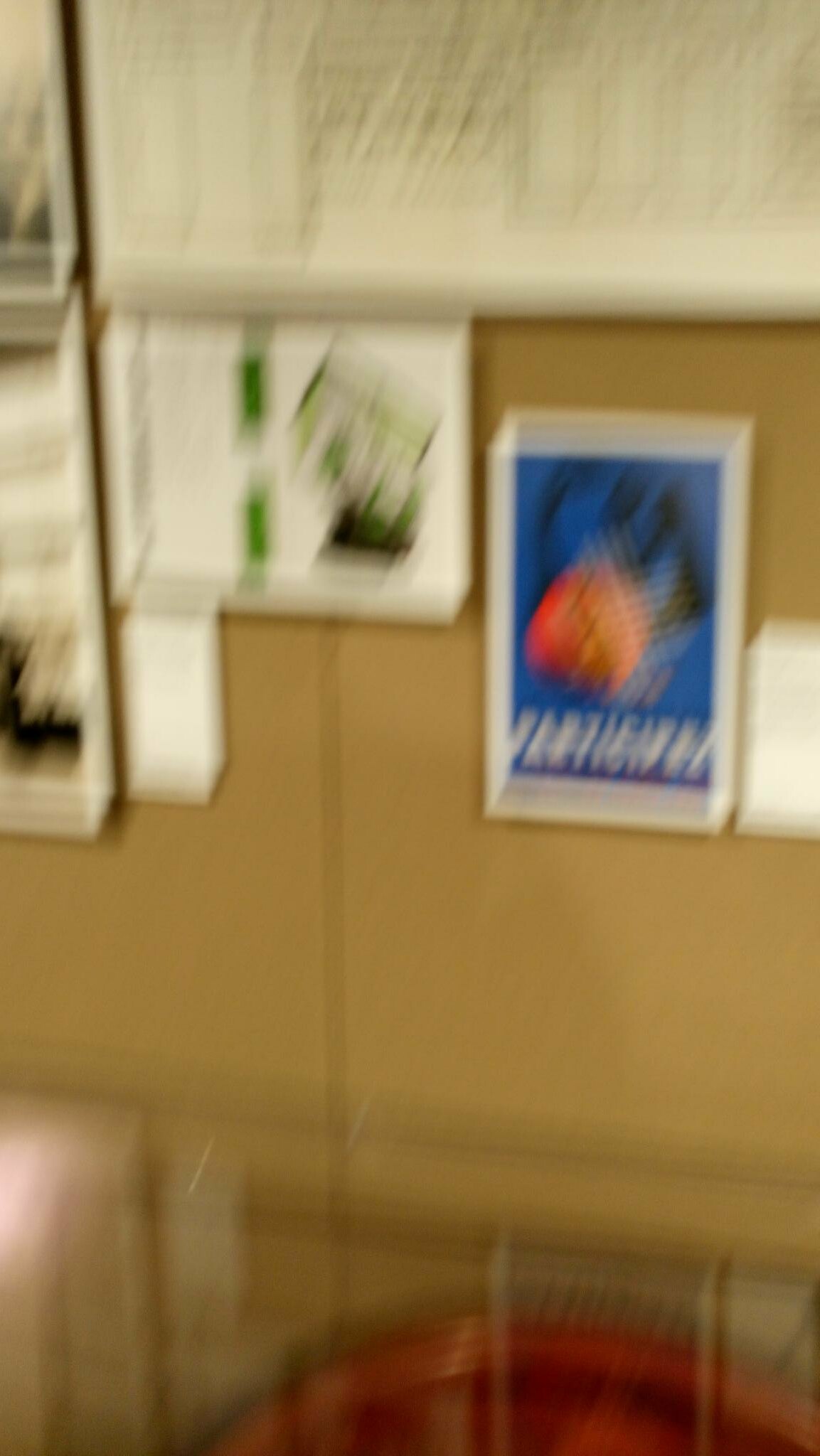This image is extremely blurry, making it difficult to discern specific details. It appears to show a cork bulletin board with various flyers and notices pinned to it. The background of the board is tan, indicating the typical cork material. On the left side, there is a prominent blue flyer with a white trim. Although the text is obscured due to the blurriness, there are black words with a reddish image beneath them and additional white words crossing the flyer. Further to the right, another flyer can be seen; this one is white with green lines down the middle and seems to feature an image on its left side. Towards the bottom left-hand corner of the image, there is a partial view of a red circle with some brown or green hues behind it. Additionally, scattered faint patches of yellow and beige lines can be observed around the board, although their purpose or content is unclear.